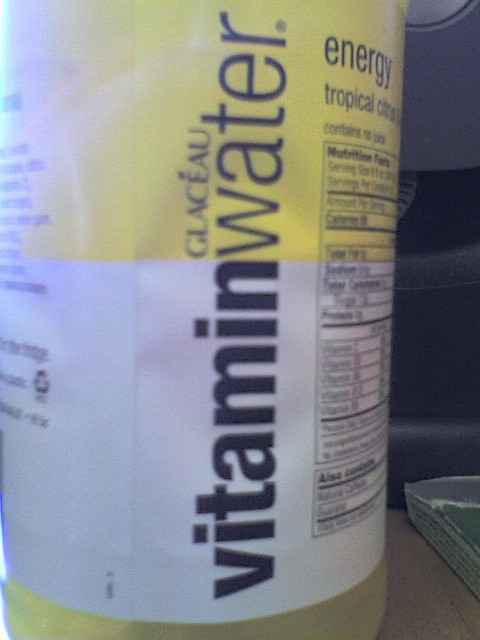This is a detailed colour photograph of a vitamin water bottle captured in a close-up shot, focusing primarily on its label. The bottle sits on a brown surface, and on the right side, a silver rectangular object is partially visible. The label itself has a distinctive design with an almost equal distribution of pale yellow at the top and white at the bottom, with a yellow band near the base. Vertically along the side of the bottle, the word "glasso" can be seen, along with "vitamin water," where the word "vitamin" is bolded, and "water" is in regular font. On the top right of the label, "energy" is written in lowercase black letters, followed by "tropical citrus," with the rest of the phrase unreadable due to small text size. The label also includes the phrase "contains no juice" and features a rectangular nutritional label with a black border, listing various vitamins, minerals, serving size, and total fat content. The left-hand side of the label has additional text that is blurred and not readable due to lighting. The background shows gradient shades of grey, indicating a wall behind the bottle.